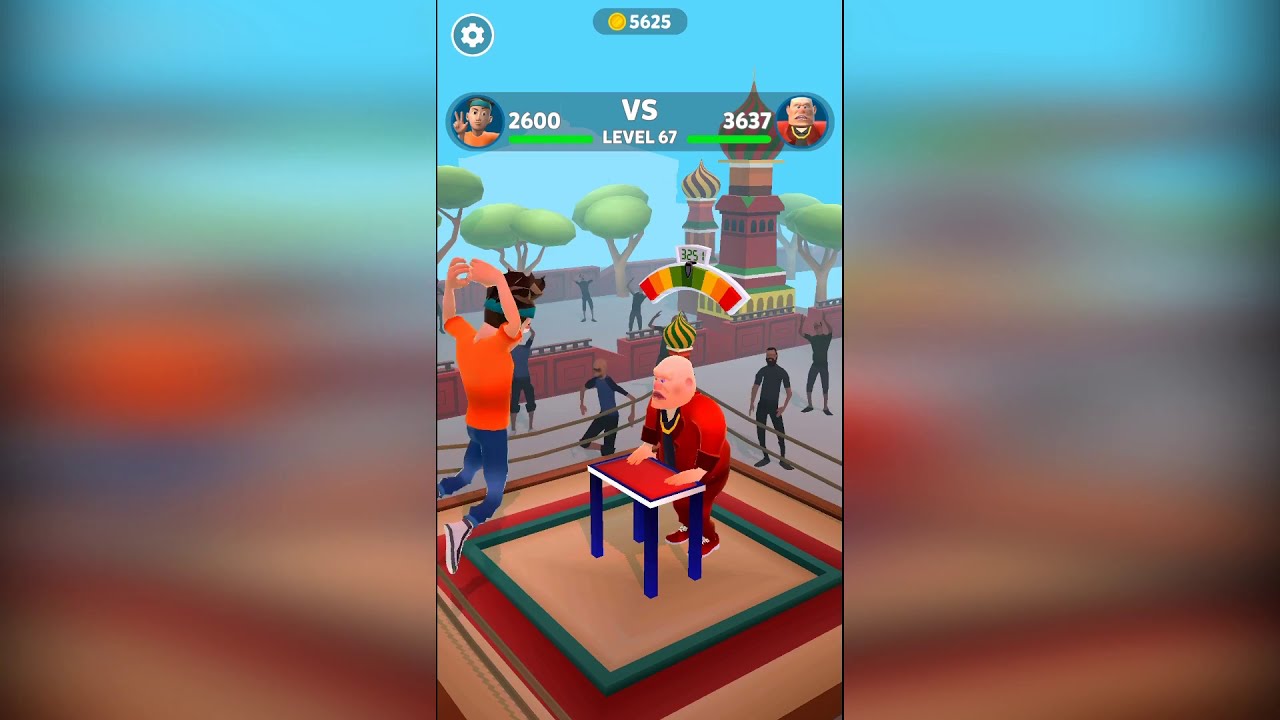The image depicts a vibrant and dynamic battle scene from a mobile video game, set within a digital world. The central focus is a rectangular in-game screenshot that includes, at its heart, a wrestling or boxing ring, dominated by a blue and red table. In this ring, a bald man with a mustache, dressed in a red shirt and white shoes, stands with his hands on the table. Opposing him is a younger, fit individual, captured in mid-air as he leaps towards the older man. The young man wears a short-sleeved orange t-shirt, blue jeans, and red shoes, with a striking blue aqua headband securing his wavy black hair.

In the backdrop of this intense confrontation, smaller, shadowy figures can be seen cheering, set against a scene that includes various elements like light and dark green trees and iconic Russian architectural structures resembling Moscow's basilicas. Above the ring, the scoreboard features circular portraits of the combatants, labeling the man in orange with a score of 2600 and the man in red with 3637 points, connected by a "VS" marker indicating a level 67 battle. Additionally, a coin count of 5625 is displayed prominently.

The overall color palette of the image is rich with vibrancy, from the protagonists' clothing—orange, red, and blue—to the tan, aqua, and red hues of the ring floor, and the blend of background colors such as red walls and blue sky. The image effectively captures the excitement and competitive spirit of a video game showdown within a vividly rendered, albeit primitively 3D, digital arena.